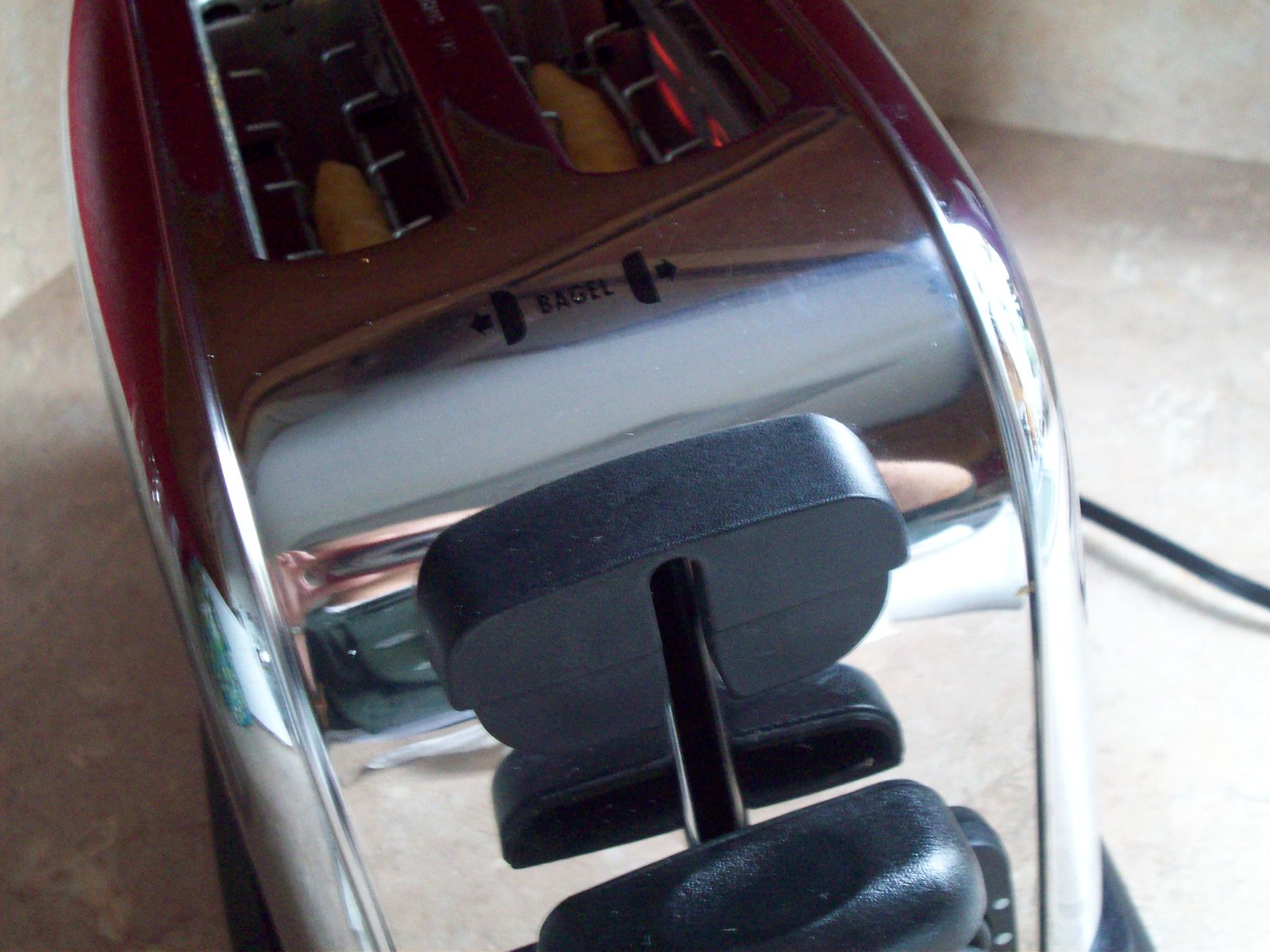This is a detailed, close-up landscape photograph of a reflective, chrome silver toaster sitting on a light grey or beige marble-patterned countertop positioned in the corner, with light walls on either side. The toaster features a black plastic handle, which is pressed down, and a black knob on the front that controls the toaster's settings. Above the two slots on its top surface, a label reads "bagel” with arrows pointing outward, indicating the correct orientation for bagels. Inside the toaster, which is currently on and heating, two bread-like items, possibly toaster strudels or bread, are visible. The red glow of the heating elements is prominent in the right slot, signifying that toasting is in progress. On the right side of the toaster, a black cord is seen trailing away. Additionally, the highly polished surface of the toaster reflects the image of the person taking the photograph using a phone.